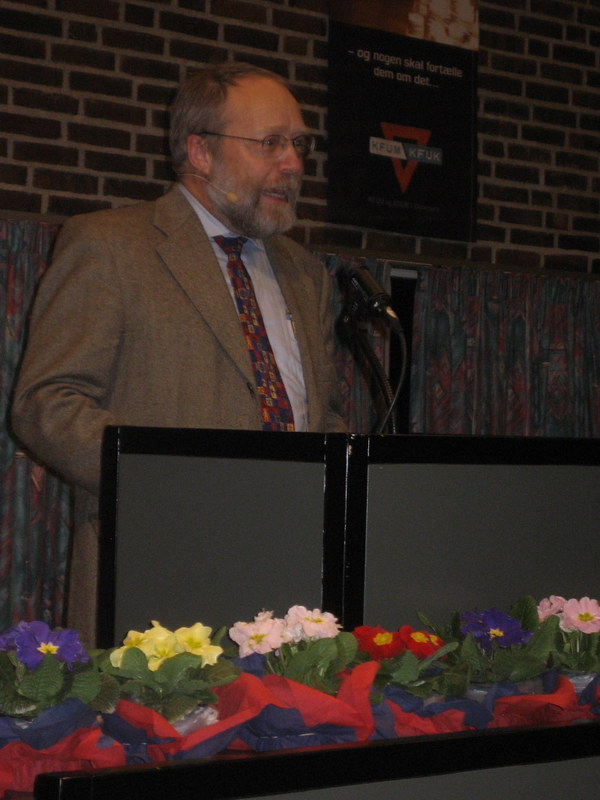The photograph captures a man standing at a podium adorned with multicolored flowers and speaking into a microphone. The podium, gray with black trim, is surrounded by an array of flowers, including purple, yellow, pink, and red blooms, each featuring green leaves and vibrant yellow centers. Behind the man is a red brick wall with a black sign displaying foreign text. A prominent red upside-down triangle symbol is visible. The man, who sports a gray and salt-and-pepper beard and black-framed glasses, is dressed in a beige jacket over a white collared shirt and a multicolored tie. He speaks into a microphone on the podium and has another microphone attached to the side of his face. The scene is further characterized by the background details, including a gray and black trim wall and hints of red and green curtains. The foreign text on the sign adds an intriguing element to the setting.